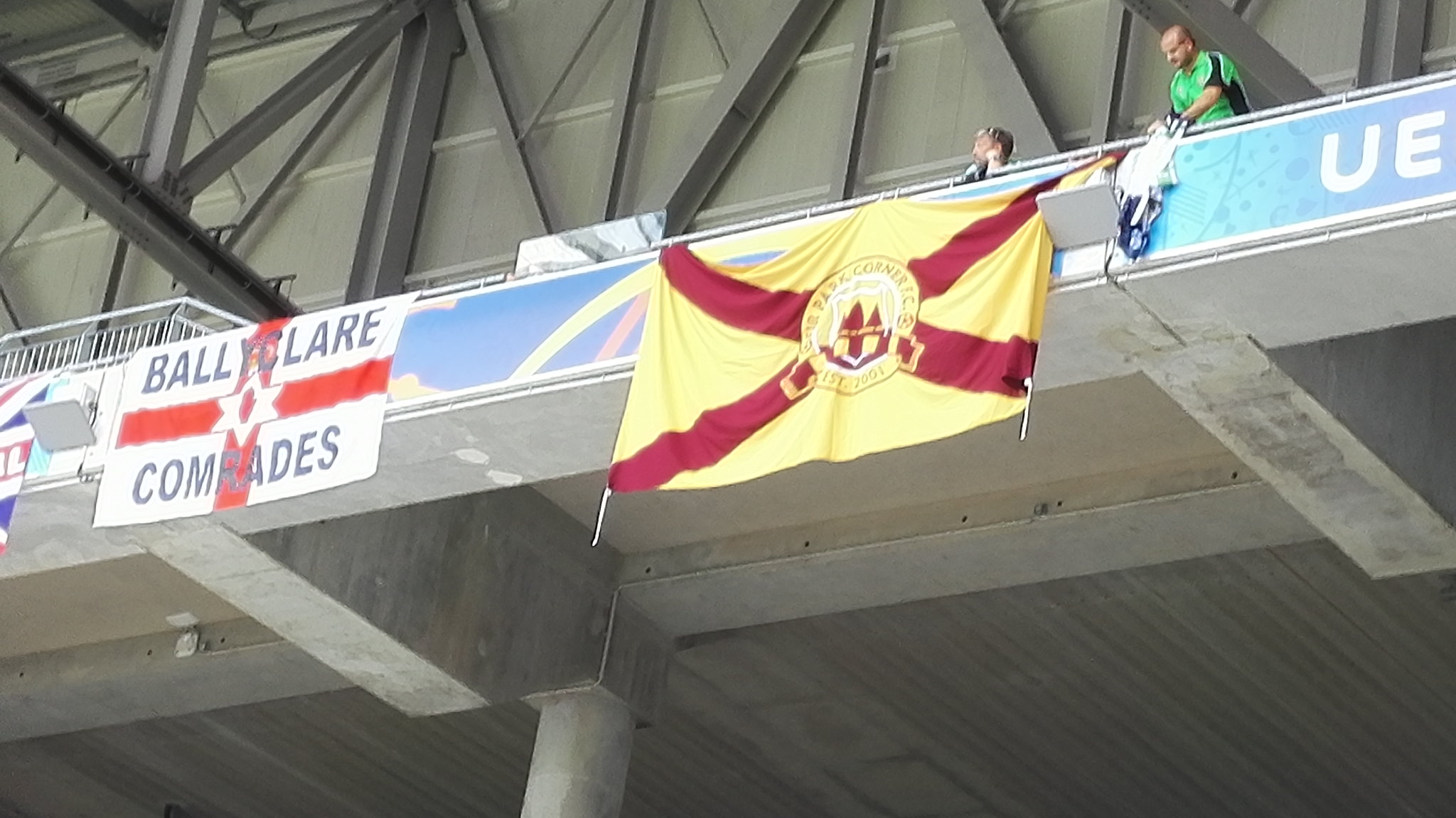The photograph appears to be taken inside a large stadium or arena. In the lower part of the image, the underside of a concrete upper level with metal girders is visible, supporting the structure above. Pillars hold up this level, and a flag prominently hangs from it, displaying a red X on a yellow background with text that seems to read "Park... Park Garner or Ghosts," and "Established 2021." Further to the left, another flag is seen with the words "Bailey Claire Comrades," featuring a star and a red cross on a white background. Two men are positioned on the far right side; one, wearing green and black, appears to be unveiling another flag. Over the entire scene, logos and text are partially visible, including one that reads "UE." The colors in the image include silver, gray, blue, white, green, black, red, and yellow, contributing to the indoor ambiance of the arena.